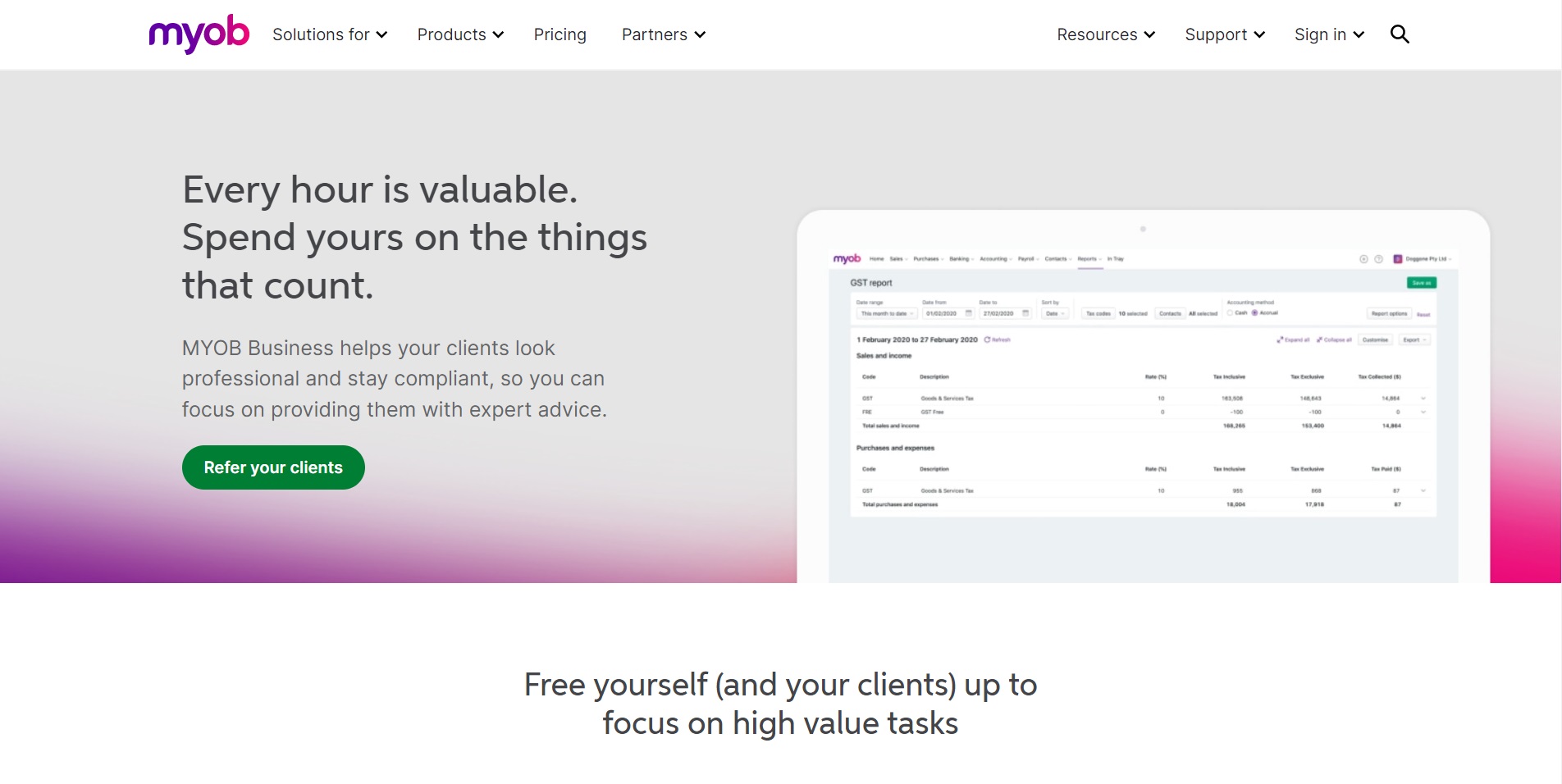The screenshot is displayed in landscape mode, with the bottom section featuring a white background. Centered at the bottom is the text, "Free yourself (and your clients) to focus on high-value tasks." In the upper right-hand corner is the MYOB logo, transitioning from purple to red, though the acronym's meaning is unclear (traditionally, it stands for "Mind Your Own Business"). 

Adjacent to the logo are navigation labels: "Solutions ▼", "Products ▼", "Pricing", "Partners ▼". Further to the right, navigation options include "Resources ▼", "Support ▼", "Sign In ▼", and a search icon.

The main content area gradually transitions from gray at the top to purple and light pink at the bottom. On the left side, the gray background features the text: "Every hour is valuable—spend yours on the things that count. MYOB Business helps your clients look professional and stay compliant, so you can focus on providing them with expert advice." Below this text is a green button labeled, "Refer your clients."

On the right side of the image is a small, difficult-to-read screenshot, presumably showing what you would get upon signing up. It appears to be a report, possibly titled "OST Report," for the period from February 1, 2020, to February 27, 2020. The report includes sales and income data, presented in a chart format, intended to help you understand how your client's business is performing.